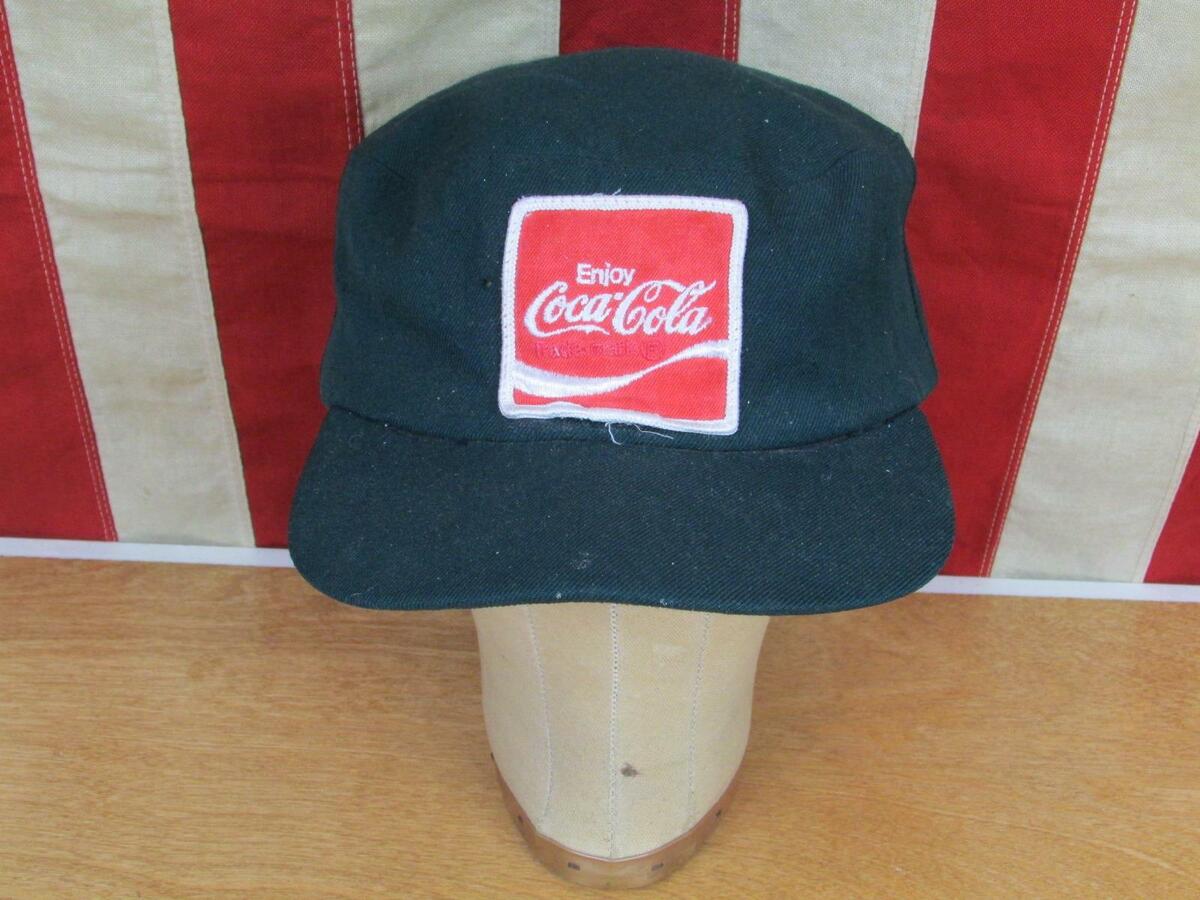The photograph features a simple but iconic black baseball cap adorned with the classic red and white square Coca-Cola logo. The logo, prominently stitched on the front, features the famous "Enjoy Coca-Cola" text in white with the distinctive curvy font and swoosh underneath. The hat appears somewhat worn, possibly covered in lint. It is positioned atop a head model meant for displaying hats or wigs. This model blends into the scene, making it difficult to see against the cap. The cap and display rest on a light, sealed yet unstained wooden shelf or table. In the background, the lower section of an American flag is visible, showcasing its vertical red and white stripes. The woven fabric of the flag, complete with white threading on the red stripes, adds a touch of patriotic ambiance to the scene.